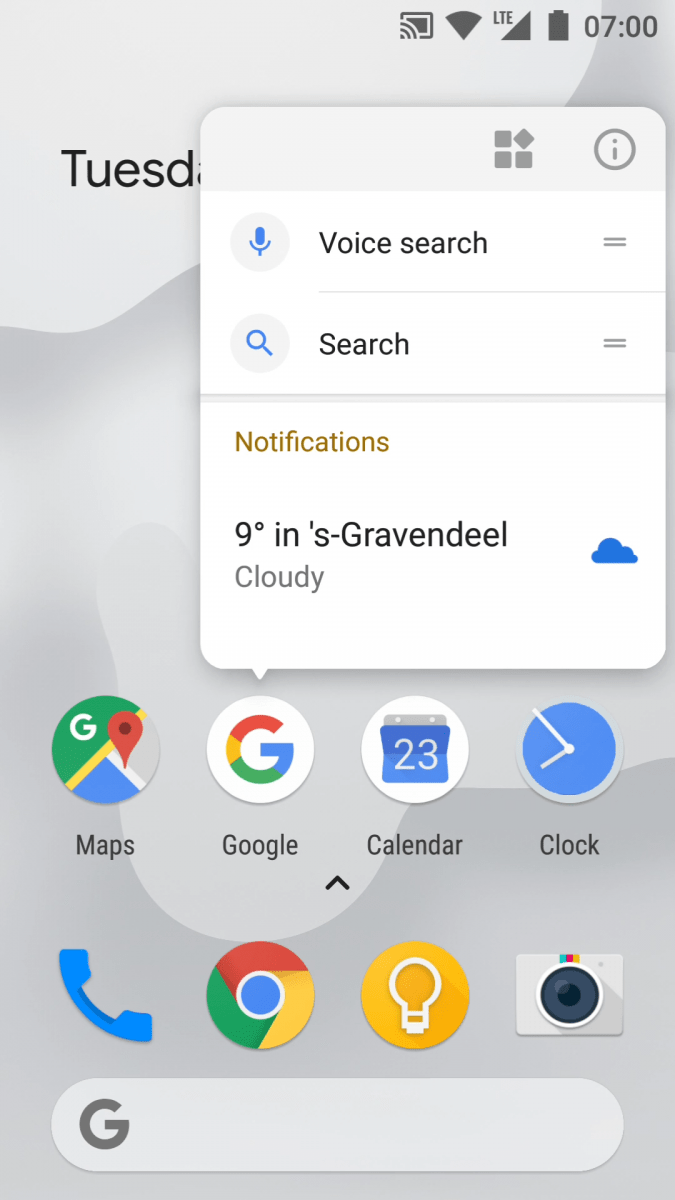The image displays a phone's home screen with a mixed gray background. In the top right corner, there are five icons: a square with three curved lines, a Wi-Fi symbol, a connection symbol, a full battery icon, and the time reading 07:00. Below this, a white square with a light gray top contains the options for voice search and a regular search bar. Underneath, "Notifications" appears in light brown text, followed by the text "9°S-GRAVENDEEL" in black, accompanied by a blue cloud icon and the word "cloudy" on the left. 

The home screen features eight apps arranged in two horizontal rows of four. The first row consists of Maps, Google, Calendar, and Clock. The second row includes a blue phone icon, Google Chrome, a yellow circle with a white light bulb, and a camera icon that is light gray with a black lens. At the bottom, there is a light gray oval with a gray "G" on the left.